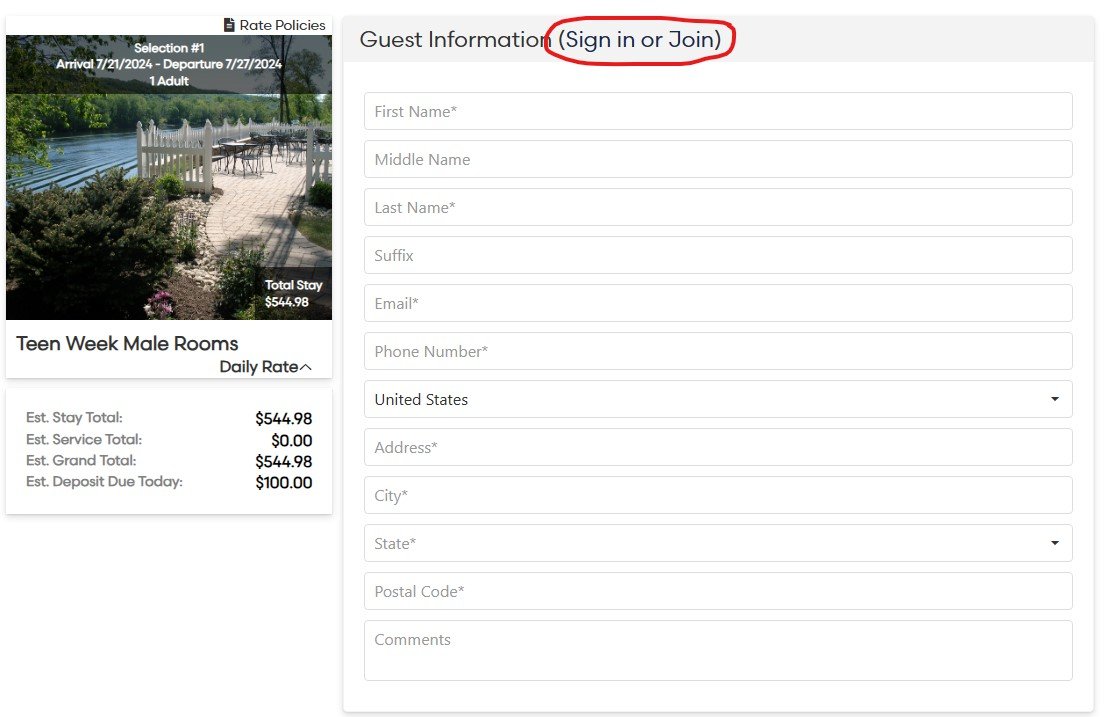This image displays a detailed booking page for a hotel or similar accommodation. On the far left, there's a picture featuring a patio with tables overlooking a tranquil body of water, such as a lake or river. The booking details indicate "Selection One: Arrival 07/21/2024 - Departure 07/27/2024" with a reservation for one adult. At the bottom right corner of this section, it mentions the total stay cost, listed as $544.98. This section also breaks down the payment details: "Teen Week Mail Rooms Daily Rate", the total estimated stay cost of $544.98, the estimated grand total of $544.98, and an estimated deposit due today of $100.

To the right of this image, there's a guest information section which prompts users to either "Sign In" or "Join", with the instructions being circled in red. The form includes fields for First Name, Middle Name, Last Name, Suffix, Email, Phone Number, Address, City, State, Postal Code, and Comments.